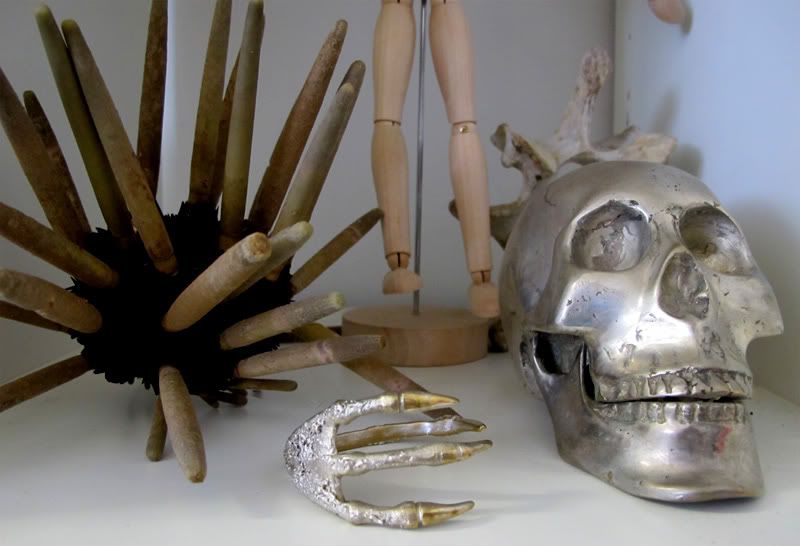The image depicts an assortment of collectible antique items arranged on a white counter against a grayish-blue background, possibly in a workshop. Dominating the right side of the photo is a detailed silver skull, with a metallic bone-like structure visible behind it. In the bottom middle, there is a tin or silverish claw. On the left side, an unusual wooden structure made of multiple sticks protruding from a central black fabric catches the eye. At the middle top, a doll or mannequin with brown legs stands upon a wooden base, supported by a silver stem. Overlaid text on the image, part of a watermark, reads "photobucket protect more of your memories for less," indicating the image's source as an advertisement for a photo hosting website. The colors in the scene vary from egg white and tan to metallic silver, adding to the eclectic and intricate appearance of the setting.